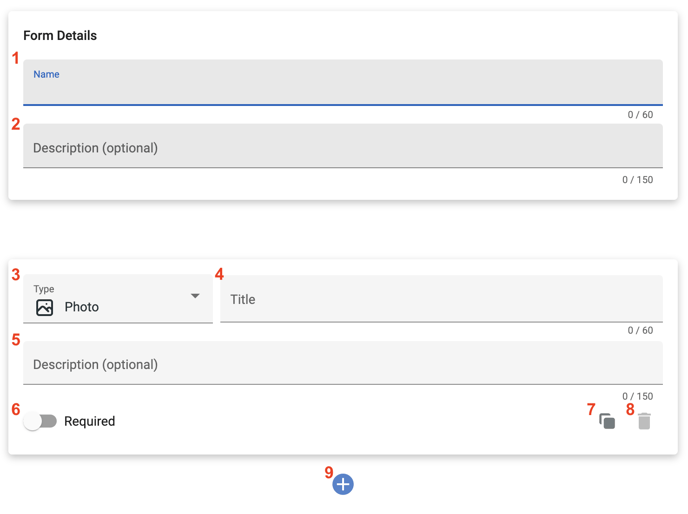The image depicts a minimalistic, text-based interface page designed for configuring a form. The background is entirely white, offering a clean and straightforward aesthetic. 

At the top left corner, there is a section labeled "Form Details" in navy blue text. This section spans the width of the page and occupies about half of the screenshot's upper portion. The section includes two lines, each beginning with a red line number. The first line is labeled "Name" and includes a pale blue delineated text box for input. The second line is labeled "Description (optional)" and is accompanied by another pale blue text box for input.

Following a white margin, the lower half of the page contains another horizontally rectangular section meant for photo configuration and additional form details. This section is divided into multiple lines:

1. Line three, numbered in red, labeled "Photo" with a downward arrow icon indicating a dropdown or file selection option.
2. Line four, numbered in red, labeled "Title" with a pale blue text box.
3. Line five, numbered in red, labeled "Description (optional)" with another pale blue text box.
4. Line six, numbered in red, features a slider set to "Required."

In the lower right corner, red numbers seven and eight denote options potentially indicating different pages or files available for selection.

At the very bottom center of the page, marked with a red number nine, lies a blue circle with a white plus sign, suggesting an action to add a new item or section.